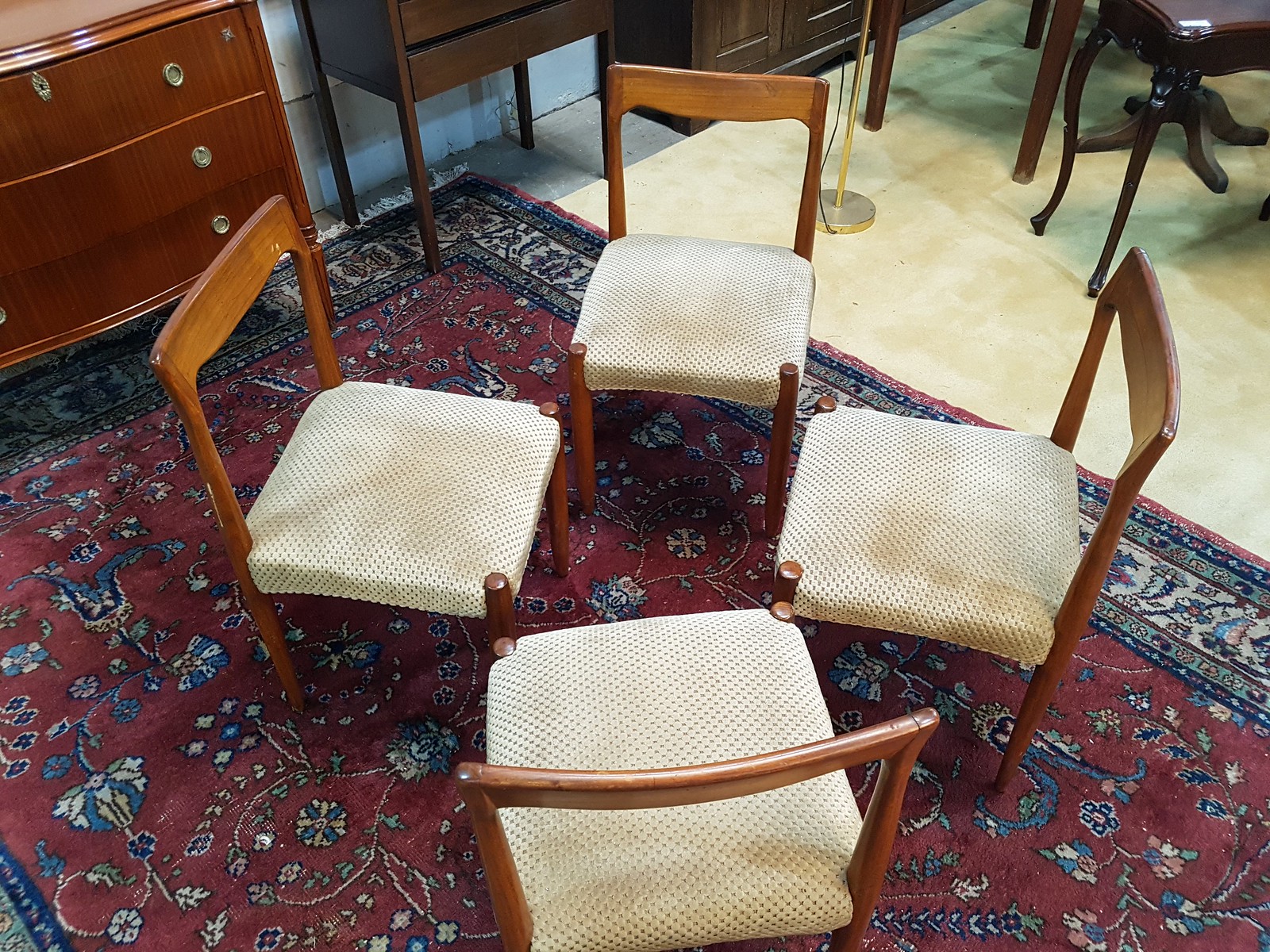The digital photograph appears to be taken in an office setting or possibly a furniture store. Dominating the center of the image are four chairs arranged in a diamond or square shape, resembling a setting for a meeting. These chairs have white wooden frames with creamy white seat cushions. They rest on a large, intricately designed area rug, predominantly red with floral patterns in white, blue, and yellow. 

In the background, starting from the upper right, there is a stylish brown chest of drawers with three metal-handled drawers visible, adjacent to a white wall. To the left of this chest, there is a darker brown cabinet. The floor transitions from the patterned rug to either white tiles or a white carpet. A portion of a silver lamp base can be seen on this floor. The top-right corner of the photograph shows a piece of very dark black furniture, completing the backdrop of the setting.